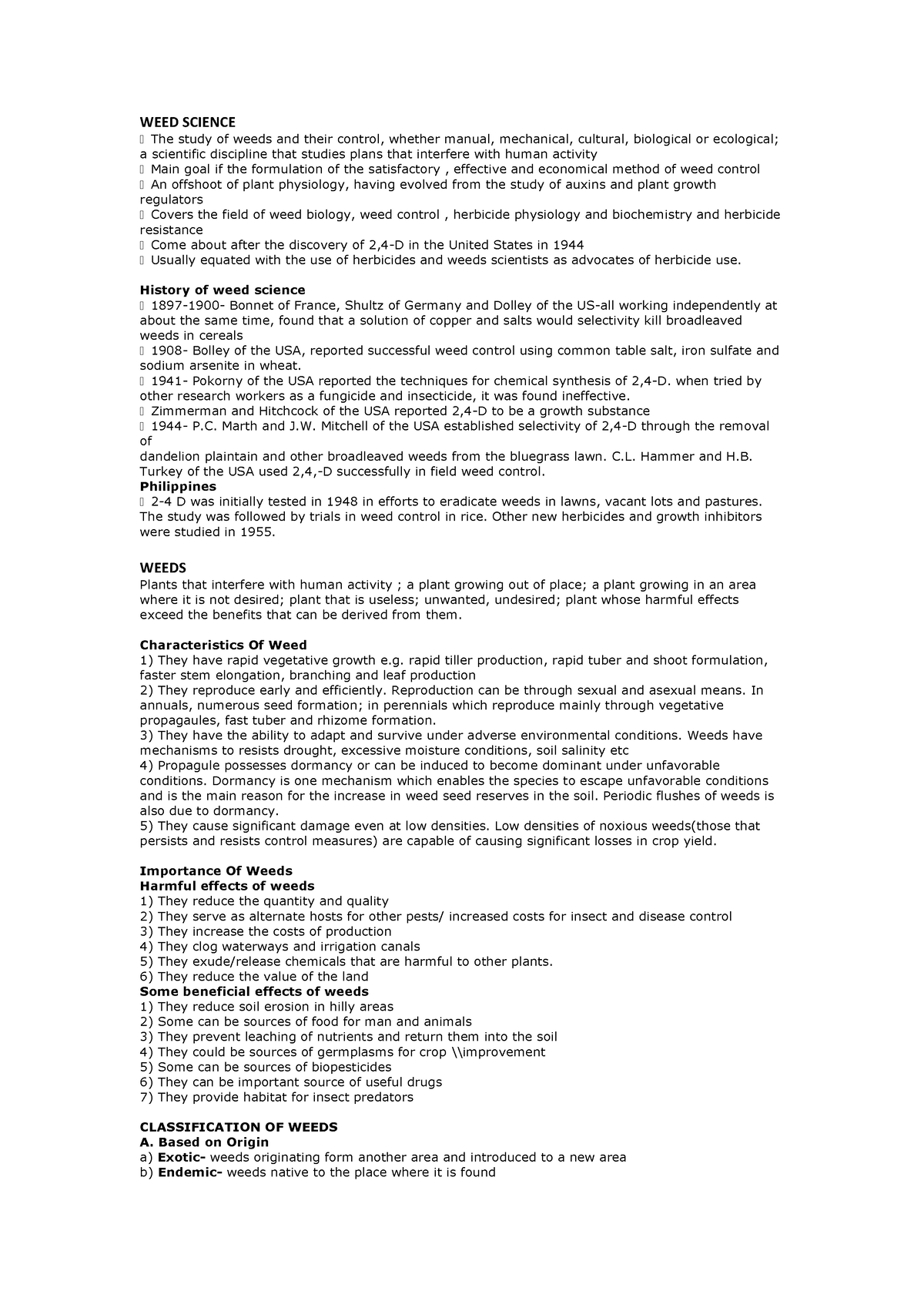The image features a detailed textual background split into black and white sections that meticulously outlines the field of weed science. 

"**Weed Science: A Comprehensive Overview**

Weed Science, the study of weeds and their control methods—be it manual, mechanical, cultural, biological, or ecological—emerges as a significant scientific discipline. This field focuses on plants that interfere with human activities, aiming to develop satisfactory, effective, and economical weed control techniques. Stemming from the study of auxins and plant growth regulators, Weed Science now encompasses weed biology, weed control, herbicide physiology and biochemistry, with herbicide resistance research gaining momentum post the discovery of 2,4-D in the United States in 1944. Historically equated with the use of herbicides, weed scientists often advocate for their use due to effective outcomes.

**Key Historical Developments: 1897 - 1990**

- **1897-1990:** Pioneering figures such as Bonnet of France, Schwartz of Germany, and Dahlia of the USA independently discovered that a copper and salts solution was effective in killing broadleaf weeds in cereals.
- **1908:** Bali of the USA reported using common table salt, iron sulfate, and sodium arsenite for successful weed control.
- **1941:** Poconee of the USA synthesized 2,4-D, though initial research found it ineffective as a fungicide or insecticide.
- **1944:** P.C. Moff and J.W. Mitchell of the USA demonstrated the selectivity of 2,4-D by successfully removing dandelions, plantains, and other broadleaf weeds from bluegrass lawns.
- **1944:** C.L. Hemmer and H.B. Turkey of the USA utilized 2,4-D effectively for controlling feed weeds.

This exploratory journey of Weed Science showcases its evolution from basic plant physiology to a robust discipline essential for agricultural and environmental management."